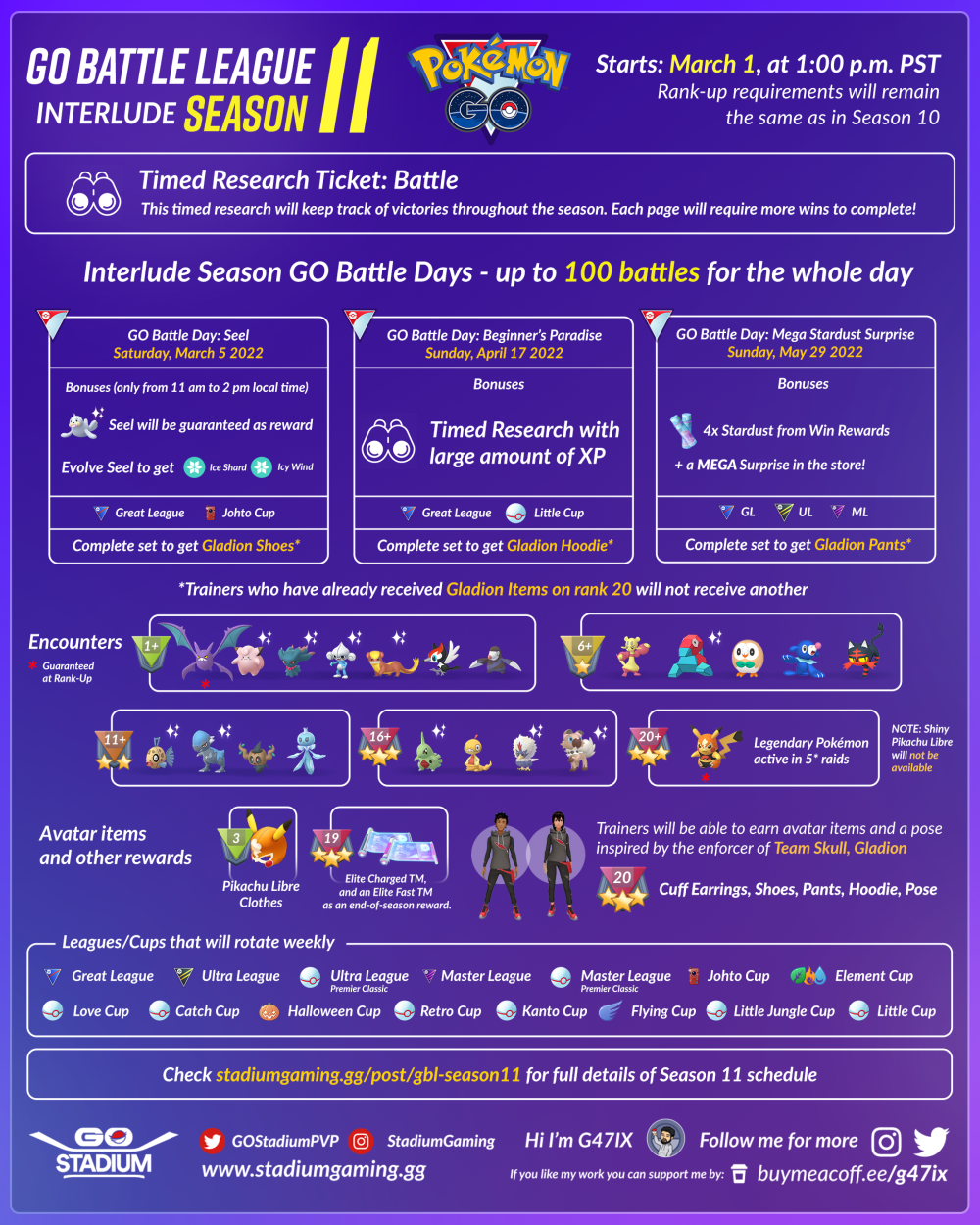The image displays a promotional poster for the Go Battle League Interlude Season 11 in Pokémon Go. To the left, the text "Go Battle League Interlude Season 11" is prominently featured, with "Season 11" highlighted in yellow and "Go Battle League Interlude" in white. Both "Go Battle League" and "Season 11" are in bold fonts to emphasize their importance.

On the right side of the image, the number "11" appears in yellow, extending vertically from top to bottom. At the top center of the poster, the Pokémon Go logo is displayed. The logo consists of an upside-down triangle with "Go" at the bottom, a Pokéstop symbol to the right, and "Pokémon" in yellow at the top, while "Go" is in dark blue.

Beneath the logo, the text "Start March 1st at 1pm PST" is shown, followed by a notice that "Rank Up Requirements will remain the same as in Season 10." Below this, in an overlay box, the text "Time to Research Ticket Battle" is noted. Additionally, it mentions that on Go Battle Day, players can participate in up to 100 battles throughout the day.

Further down, key dates for Go Battle Day events are listed. The first event, "Go Battle Day Seals," is scheduled for March 5th, 2022. In the middle, "Go Battle Day Beginner's Paradise" is set for April 17th, 2022. Another event, "Go Battle Day Mega-Style Surprise," will take place on April 29th, 2022. It is also specified that trainers who have already received Gladeon items at Rank 20 will not receive them again.

On the left side of the image, there is a box featuring images of 7 Pokémon, with additional groups of 6 and 5 Pokémon. Below this, more details about character avatar clothes and rank items are provided.

At the bottom, certain leagues and a URL are listed. The background of the image transitions from an indigo color at the top left to a lighter purple at the bottom right, adding a gradient effect.